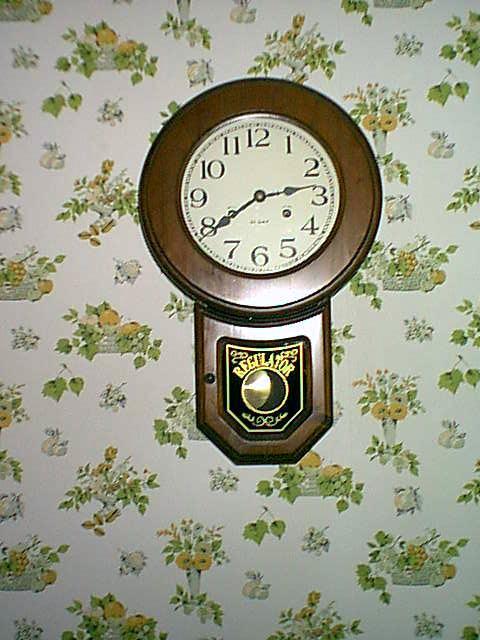A detailed photograph showcases a vintage wall clock hanging on a beautifully wallpapered wall. The wallpaper features an elegant design of yellow and white flowers interspersed with green leaves, arranged in various vases. The predominant color of the wallpaper is white, providing a bright backdrop for the intricate floral patterns.

The classic clock boasts a rich brown wooden frame. Beneath the clock face, there's a section that reads "Regulator" in gold letters, adding a touch of sophistication. This section also includes a small plaque and a tiny knob on the left side, suggesting the presence of a small door beneath the clock, possibly for accessing the pendulum or making adjustments.

The clock face itself is pristine white with bold black numerals and sleek black hands, currently indicating the time as 2:39. A light source illuminates the clock, casting a gentle glow on the upper face and the lower base, highlighting the fine craftsmanship of the timepiece.